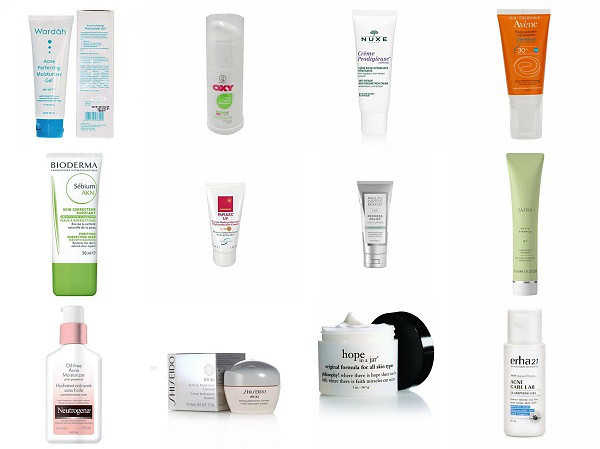This image is a meticulous compilation of 12 real-life cosmetic products, seamlessly amalgamated to form a cohesive visual display. It is important to note that each product retains its individual photographic clarity, organized in a structured grid formation. Here’s a detailed breakdown of the composition:

### Top Row (Left to Right):
1. **WADA Acne Moisturizer Gel**: A white tube topped with a blue lid. The image showcases both the front and the reverse side of the tube, providing a comprehensive view.
2. **Oxy**: This product features "Oxy" in bold red letters on a white tube, accompanied by a green leaf-like shape below the text. The writing is not entirely legible, but the design elements are clear.
3. **NUX**: A white tube positioned upright, labeled in French with "crème" partially visible. The details are somewhat obscured, but the elegance of the packaging stands out.
4. **Avene**: An orange and white tube also standing on its end. While the specific details on the tube are indistinguishable, it likely pertains to skin care, consistent with Avene’s branding.

### Middle Row (Left to Right):
1. **Bioderma**: This product is identifiable by its flattened tube and green cap. The label reads "Sebum AKN," hinting at its skincare purpose and possibly indicating a non-English language.
2. Another small white tube with a red square marking. Despite the difficulty in reading the fine print, the minimalist design catches the eye.
3. A sleek, small silver tube, devoid of readable text but adding a metallic sheen to the assortment.
4. A long, slender green tube with a white cap, also standing on its end. The specifics are unreadable, but it follows the aesthetic of a moisturizing product.

### Bottom Row (Left to Right):
1. **Neutrogena**: Featured in a white and pink bottle with a prominent pump dispenser. The black Neutrogena logo contrasts sharply against the bottle, adding a touch of distinction.
2. **Shiseido**: This high-end cream is accompanied by its elegant silver box to the left. While the product details remain unseen, the luxury branding of Shiseido is unmistakable.
3. **Hope in a Jar**: An open jar showcasing its white cream contents, the name "Hope" clearly etched on the jar. The black lid rests adjacent, reaffirming the product's identity.
4. **Erhatz**: A white and blue container standing upright with its lid securely in place. The label "Erhatz" provides limited context but suggests a cosmetic or skincare solution.

Each product in the image is uniquely positioned and visually distinct, contributing to a harmonious yet detailed display of diverse cosmetic items.